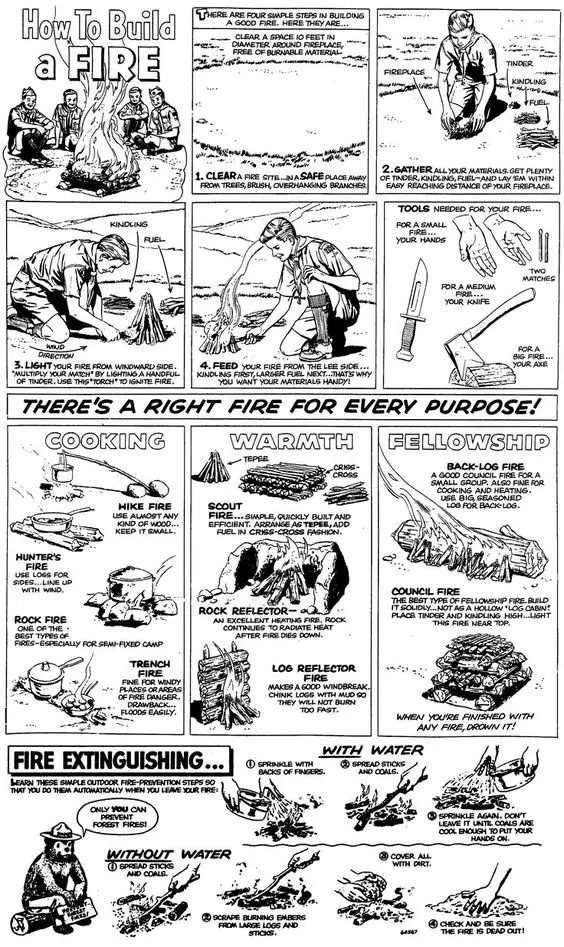The image is a detailed instructional comic cartoon from the 1950s on how to build and manage a fire, presented in a grid format. At the top, the comic starts with a large box captioned "How to Build a Fire" in bold, outlining letters. Underneath, in three successive rows of square boxes, it shows a young boy, possibly a Boy Scout, illustrating the step-by-step process of building a fire. The steps include gathering firewood, preparing the fire structure, igniting it, and feeding it to a sustainable burn. 

A mid-section horizontal banner reads, "There's a right fire for every purpose!" Below this banner are three vertical rectangular boxes depicting the fires used for cooking, warmth, and fellowship, each with explanatory illustrations and accompanying text. These sections highlight the diverse uses of a fire in outdoor settings. 

At the bottom half of the image, there's a section titled "Fire Extinguishing," prominently underlined. This section illustrates methods for putting out fires using and without using water, represented by seven images in two rows—three images labeled "with water" at the top (with "with" underlined) and four images labeled "without water" at the bottom (with "without" underlined). 

In the bottom left corner, Smokey the Bear, wearing his ranger hat, sits on a log holding a piece of paper with a speech bubble saying, "Only YOU can prevent forest fires," emphasizing the importance of fire safety.